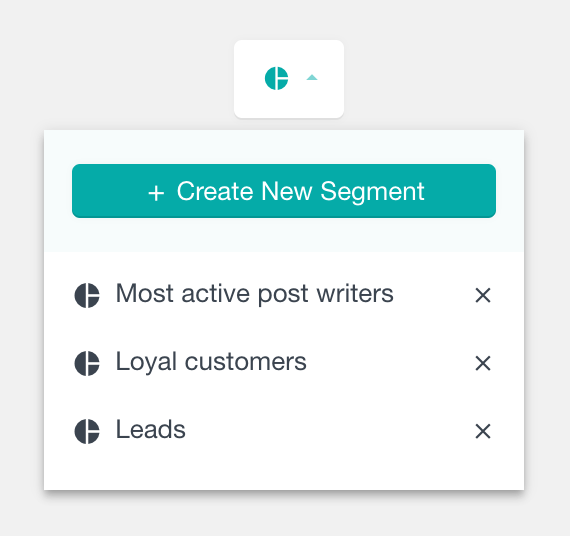The page features a minimalistic design with a light gray background. At the top center of the page, there is a white rectangle containing a blue icon. The icon is a circle divided by a vertical line, splitting it into distinct sections that resemble a Pac-Man shape. Beside this icon is an upward-pointing blue arrow.

Below this section, against the gray background, there's another white rectangle. This rectangle features a blue header bar with a centered white plus sign and the words "Create New Segment" in white text.

Beneath this, three sections are listed vertically, each with a black version of the same circle icon used earlier. The first section is titled "Most Active Post Writers" and ends with an 'X' on the right. The second section is "Loyal Customers," also ending with an 'X'. The final section is "Leads," again with an 'X' on the right.

Each of these elements contributes to a clean, organized layout that clearly distinguishes between the various segments on the page.